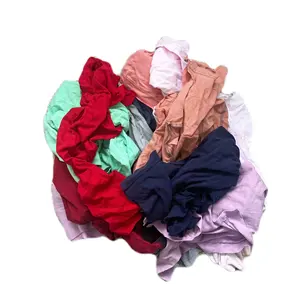In the center of the image, against a stark white background, is a disorganized pile of clothing, creating a textured, multicolored heap. The clothing appears crumpled and lacks any discernible form, making it difficult to identify specific items, though they may include shirts, pants, and potentially even socks or underwear. The lighting is good, and the image is in focus though a bit blurry to some viewers. Dominating the pile is a rich, bright ruby red fabric folded in a C shape. Nearby is a larger, muted pale mint green piece. Other colors visible in the jumble include navy blue, light lavender, peach, and white. Each piece of fabric appears to be made of relatively thin material, suggesting the clothing could mostly consist of t-shirts. Despite the clarity of the image and the vibrant array of colors, the purpose of this assortment remains unclear due to the lack of contextual cues or text.